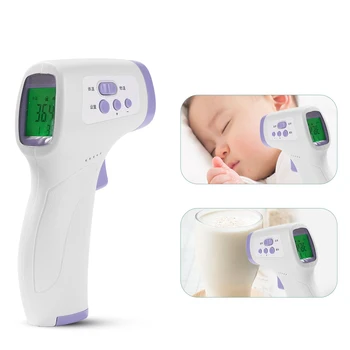The image showcases a white, handheld digital baby temperature monitor, resembling a small handgun or hairdryer, adorned with light purple, lavender accents. The primary visual element is a large illustration of the thermometer positioned on the left side, featuring a bright green digital interface displaying the temperature reading, "36.4". The device's design includes purple buttons on both sides, a purple trigger, and additional purple detailing around the screen and the sensing area.

To the right of this main image are two smaller, rounded rectangular insets demonstrating the monitor's use. The upper inset depicts a sleeping baby with pale, peachy-colored skin and brown hair, lying on its right cheek. The baby's fists are gently positioned near its mouth and nose, while the thermometer is held close to the left cheek to measure the baby's temperature.

The lower inset shows the thermometer being used to check the temperature of a clear glass of milk or formula. Both supplementary images emphasize the practicality and versatility of the thermometer for monitoring both body and liquid temperatures. The scene hints at a domestic or possibly clinical environment, stressing the importance of accurate temperature monitoring in child care.